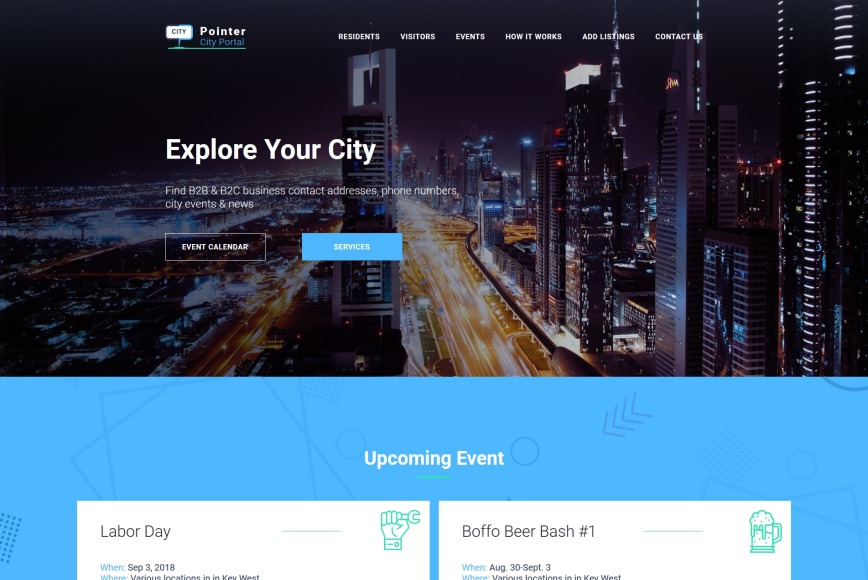A detailed caption for the provided description could be:

"The webpage features the 'City Pointer City Portal' that overlays a nighttime cityscape in the background, creating a vibrant and urban atmosphere. The top navigation bar includes sections like Residents, Visitors, Events, How It Works, Add Listings, and Contact. Beneath, the headline 'Explore Your City' invites users to find B2B and B2C business contacts, addresses, phone numbers, city events, and news. Prominent buttons for the Event Calendar and Services are also visible. The page highlights upcoming events such as Labor Day on September 3rd, 2018, and the Buffalo Beer Bash from August 30th to September 3rd. The lower portion of the page features a simple blue background adorned with circles and arrows for a dynamic design, all aimed at encouraging users to discover and engage with city activities and services."